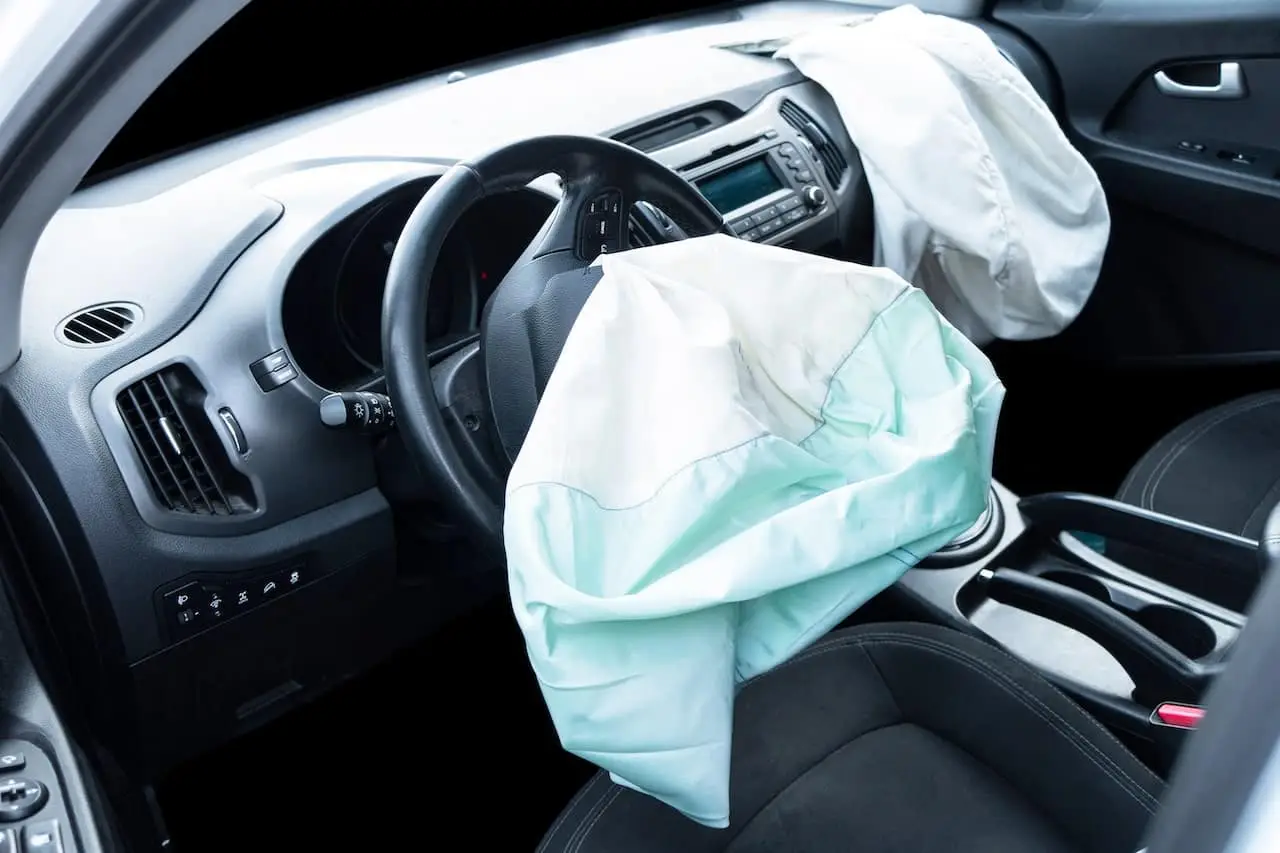The image depicts the interior of a car with both the driver's and passenger's airbags deployed. The interior, primarily dark with gray seats and gray door molding, features a black steering wheel with a white airbag partially tinged with teal blue. Similar to the driver's side, the passenger's side airbag hangs over the compartment above the glove box. The car appears to be in park with no additional damage apart from the deployed airbags. Visible details include the stereo system on the dashboard, chrome door handle on the right, and bucket seats with a central console and gearshift lever, suggesting it may be a manual transmission. Notably, the interior is exceptionally clean without the typical powder residue from airbag deployment, indicating the scene may be staged.